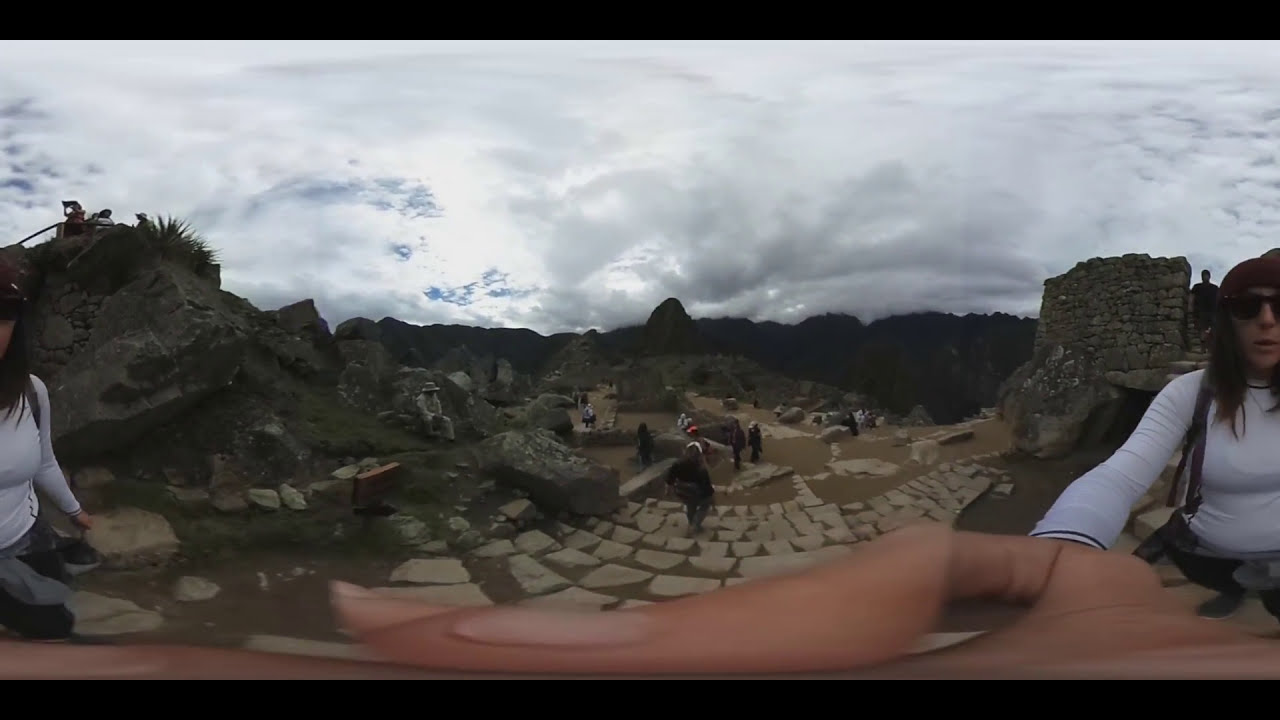This color photograph, presented in landscape orientation, depicts a popular tourist site featuring ancient ruins and stone structures. The image spans three combined photographs creating a panoramic view, framed by thin black borders at the top and bottom. The scene is set under a cloudy sky, with darkening clouds hinting at impending rain.

In the image, the same woman appears twice due to the panoramic stitching effect. She has long, dark hair draped past her shoulders, and she is dressed in a long-sleeved white top, sunglasses, and a red hat. On the left, the woman is partially visible standing beside a hillside covered with stones and sparse vegetation. On the right, she appears again, more prominent and facing the camera with her arm extended. A distorted hand, likely hers, is visible at the bottom of the frame.

The central section of the photograph captures a stone courtyard with curved, white stone steps leading downward. Several tourists are wandering around, taking in the historic ambiance of the site. In the distance, a few trees are scattered among large boulders and stone walls. The backdrop features a blue-hued mountain range, adding depth to the scene. The photograph combines elements of representational realism with a panoramic filter, providing a comprehensive and detailed view of this intriguing historical location.